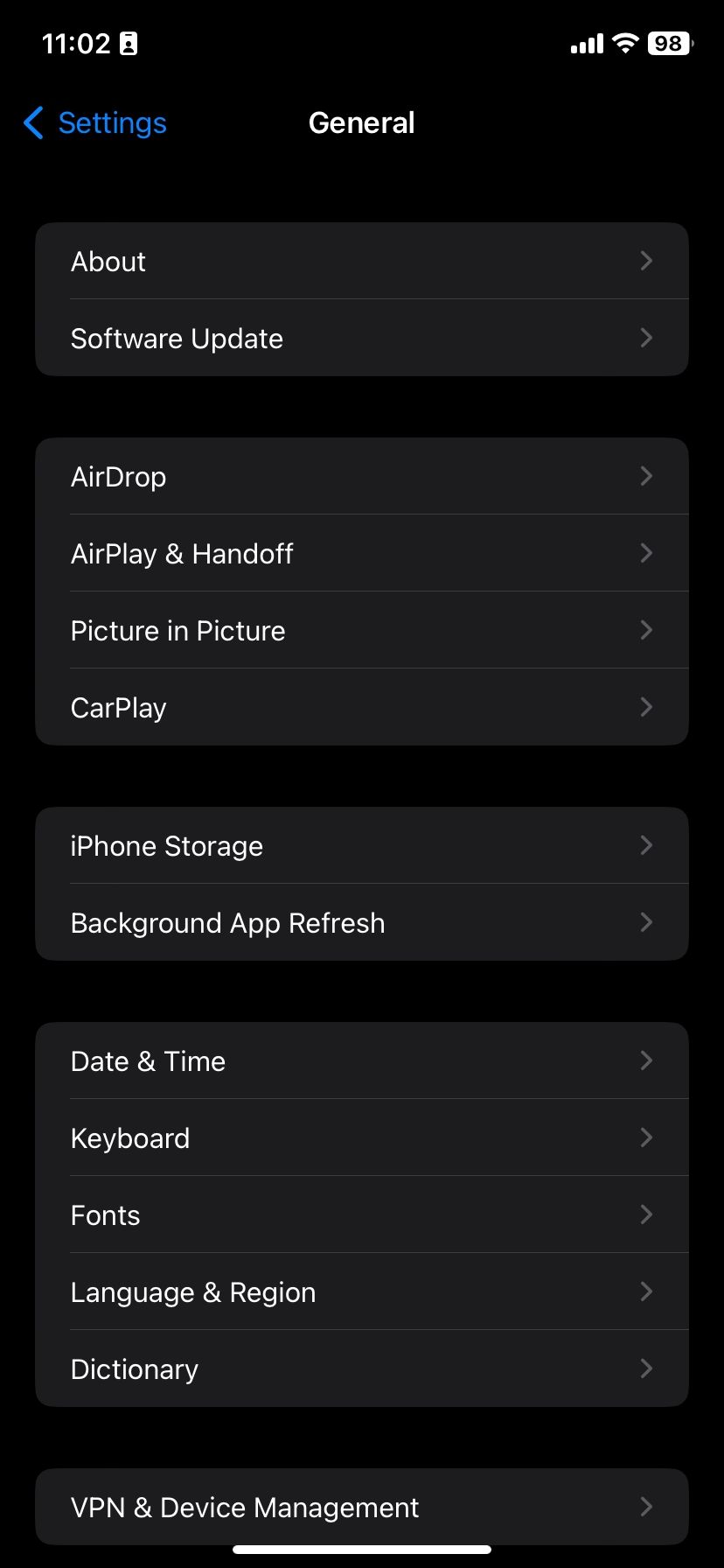In this image, we are looking at a screenshot of a cell phone screen. The upper left corner displays the time as 11:02, while the upper right corner shows a battery level of 98%, alongside Wi-Fi being on and all signal bars lit. This interface is set against a solid black background. At the very top of the screen, there is blue text that reads "Settings" followed by white text that says "General." Below this header, there is a vertical list of options that includes: "About," "Software Update," "AirDrop," "AirPlay & Handoff," "Picture in Picture," "CarPlay," "iPhone Storage," "Background App Refresh," "Date & Time," "Keyboard," "Fonts," "Language & Region," "Dictionary," and "VPN & Device Management." The neatly organized settings menu provides easy access to various configurations and features of the device.